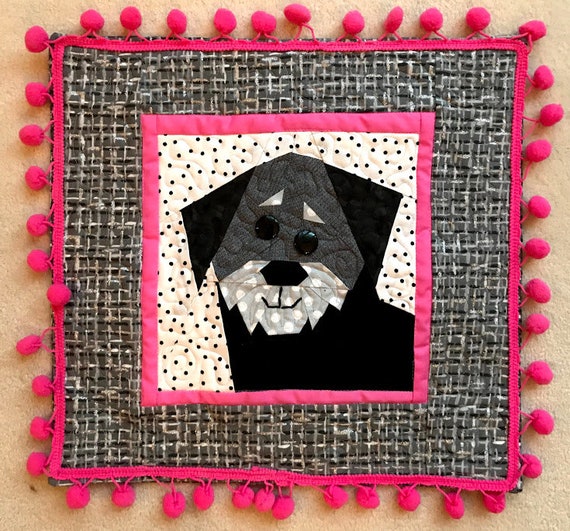This detailed image portrays a meticulously crafted square quilt that appears to double as a placemat or coaster, set against a tan background. The outermost border of the quilt is adorned with bright pink pom-poms affixed to a ribbon, providing a vivid and playful frame. Moving inward, the next section is a highly textured gray and white woven fabric, giving the piece a rich visual depth. Enclosed within this is a narrow hot pink border that further accentuates the central motif.

At the heart of the quilt is an endearing depiction of a dog, rendered in a delightful array of quilted fabrics. The dog features simple, geometric shapes: its ears are black triangles, its nose is a large black octagon, and the white triangular eyebrows add a whimsical touch. The dog’s expressive face, complete with a large black button nose and slightly askew button eyes, exudes a happy, gentle demeanor. The muzzle is crafted from grey fabric with white polka dots, providing a stark contrast to the predominantly black body. This charming canine figure is set against a white background peppered with black polka dots, enhancing the quilt's overall textural appeal.

This piece is a harmonious blend of colors defined primarily by shades of pink, black, white, and gray, and its intricate quilting suggests it was made with a sewing machine. The entire artwork rests on a tan surface, likely a table, showcasing not just the visual but also the tactile quality of the fabric art.